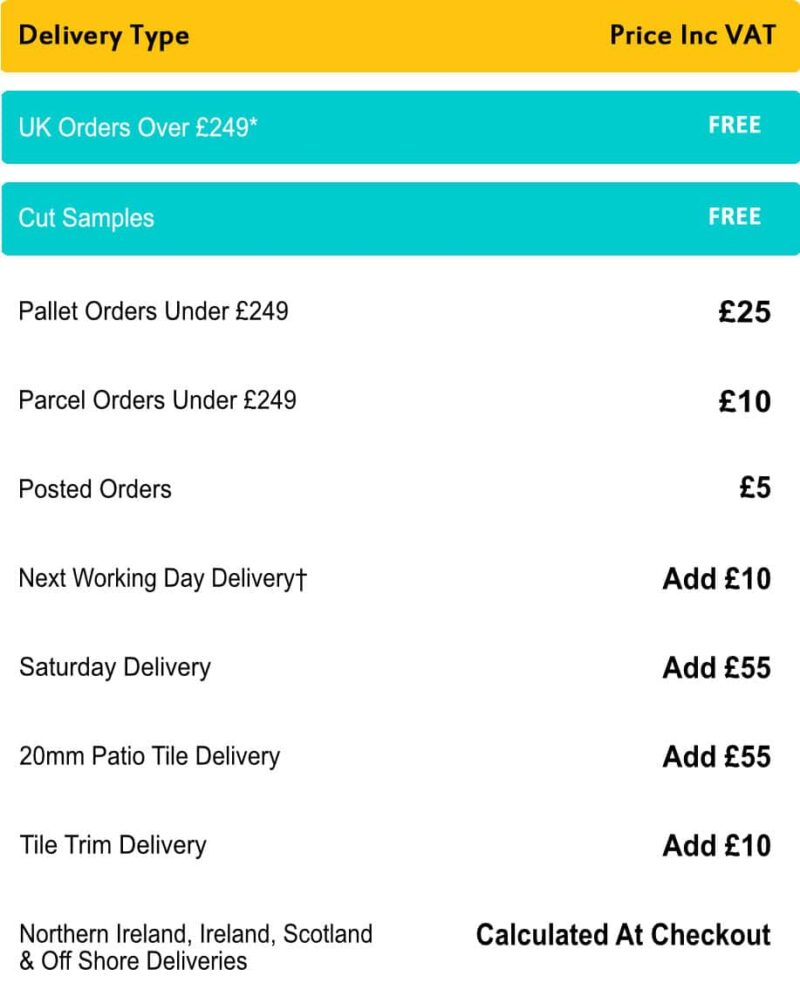### Delivery Options & Prices

---

**Delivery Type**

---

#### UK Orders Over £249*
**FREE**

---

#### Cut Samples
**FREE**

---

**Pallet Orders Under £249**  
£25

**Parcel Orders Under £249**  
£10

**Postage Orders**  
£5

---

**Next Working Day Delivery**  
✗ **add £10**

**Saturday Delivery**  
**add £55**

**20mm Patio Tile Delivery**  
**add £55**

**Tile Trim Delivery**  
**add £10**

---

**Northern Ireland, Ireland, Scotland & Offshore Deliveries**  
**Calculated at Checkout**